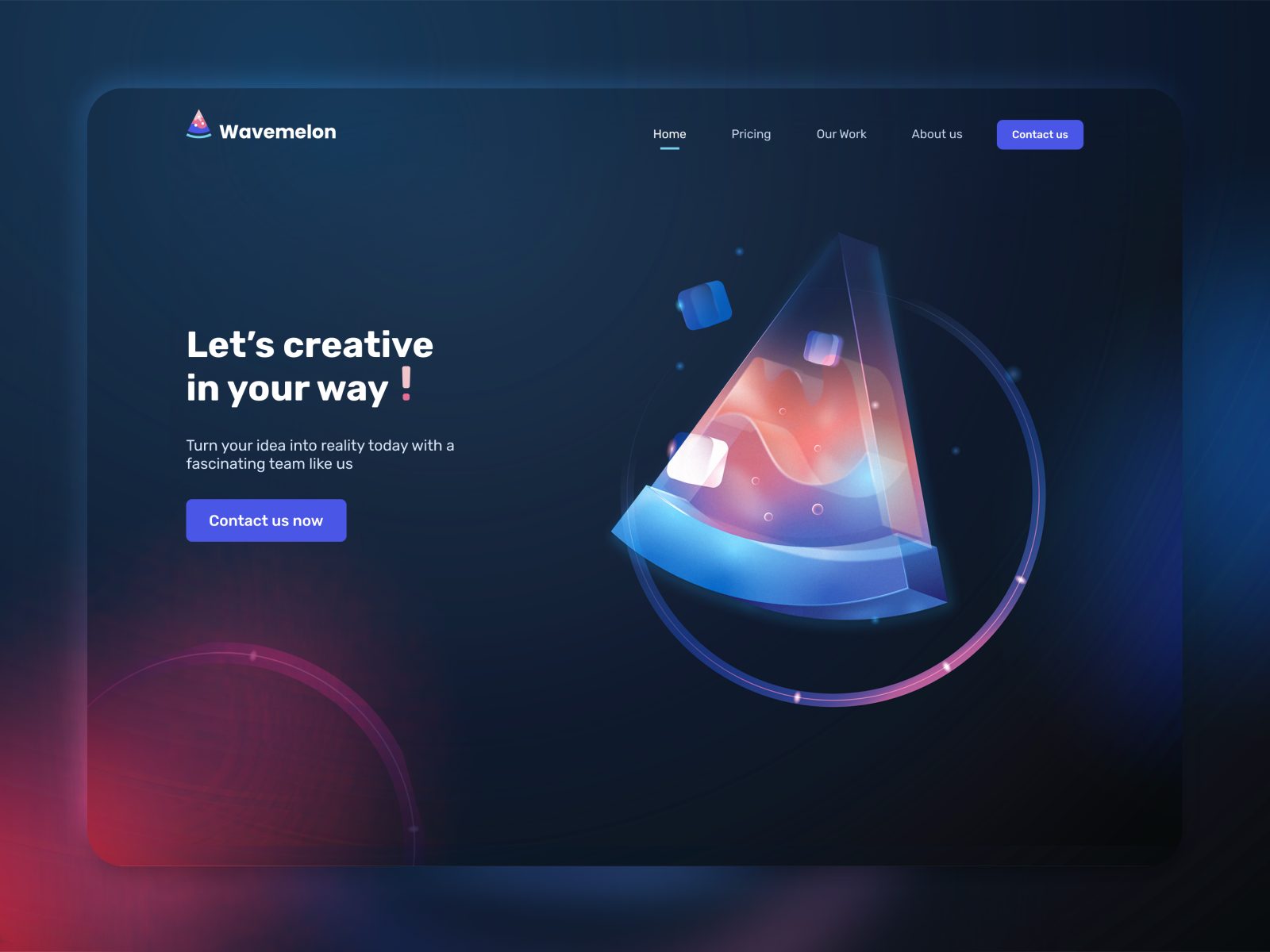The image features a gradient background that transitions from dark blue at the top to a deep purple or magenta shade at the bottom left. Moving towards the far right middle side, the colors shift into a lighter blue or purplish-blue hue, creating a unique and visually appealing blend.

In the upper left corner, the words "Wave Melon" are prominently displayed, possibly alongside an illustration that resembles a slice of watermelon, although its exact nature is uncertain. To the right of this, there is a navigation menu with several options. "Home" is highlighted with a teal-colored underline, while other menu items such as "Pricing," "Our Work," and "About Us" are listed. A blue button labeled "Contact Us" is also present in this section.

Below this menu, on the left side, large white bold letters read, "Let's Create Creative in Your Way." Underneath this slogan, in smaller, non-bold text, is the phrase, "Turn your idea into reality today with a fascinating team like us." Finally, beneath this text, there is another blue button that says, "Contact Us Now."